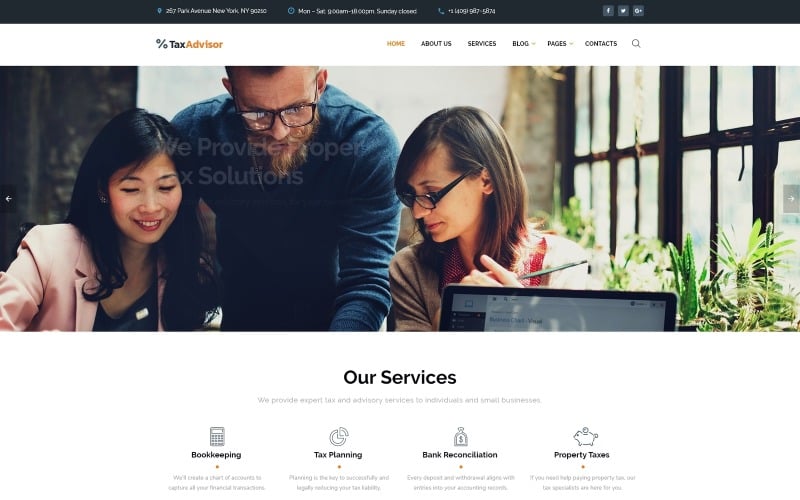The top of the image features a horizontal black bar that spans across its width. Within this bar are several sets of text and a blue symbol next to each, however, both the text and symbols are too small to discern clearly. Beneath this black bar are three gray rectangles, each containing pictures that are similarly indiscernible due to their small size.

Following these elements, the background turns white and features several textual labels. In black text, the label reads "Percent Tax." Adjacent to this, in dark yellow, are the words "Advisor" and "Home." Subsequent labels, also in black, include "About Us," "Services," "Blog," "Images," and "Contacts." A magnifying glass icon is positioned at the end of this sequence, suggesting a search function.

Continuing downward, the central section of the image showcases a picture of three people working together. One individual, a woman, has a laptop open in front of her. Superimposed on this image are words in light blue, which are faint and challenging to read due to the background. It appears to say "We provide Open X Solutions," though the exact wording remains unclear.

On the right side of the image, there is a window along with some plants, adding a touch of natural light and greenery to the setting. This composition draws attention to a collaborative and professional environment.